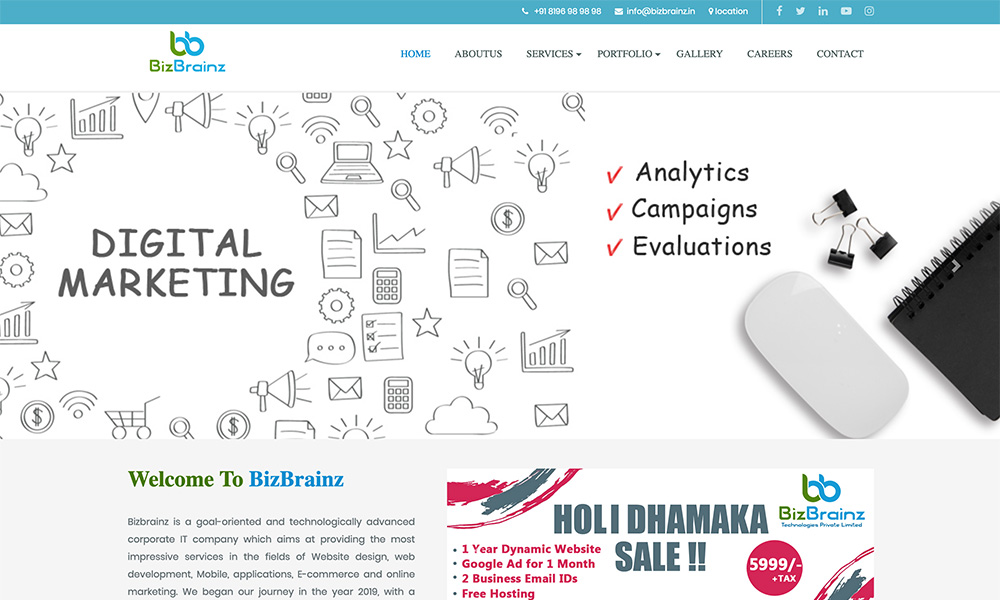This image showcases the homepage of the BizBrains website. The brand name “BizBrains” is prominently displayed in two colors: "Biz" in green and "Brains" in blue, with the text located on the upper left-hand side of the site. Above the brand name lies the company’s logo, comprised of two lowercase 'b' letters touching to form a unified symbol.

The website navigation menu includes the following options: Home, About Us, Services, Portfolio, Gallery, Careers, and Contact. The main banner of the website, positioned to the left, prominently features the text "Digital Marketing." Surrounding this text is a series of symbols arranged in a square with a central round white space. The symbols include a shopping cart, a currency sign, a laptop, a magnifying glass, and a calculator—each representing different facets of digital marketing.

To the right of the banner, there is text detailing the company's focus areas: Analytics, Campaigns, and Evaluations.